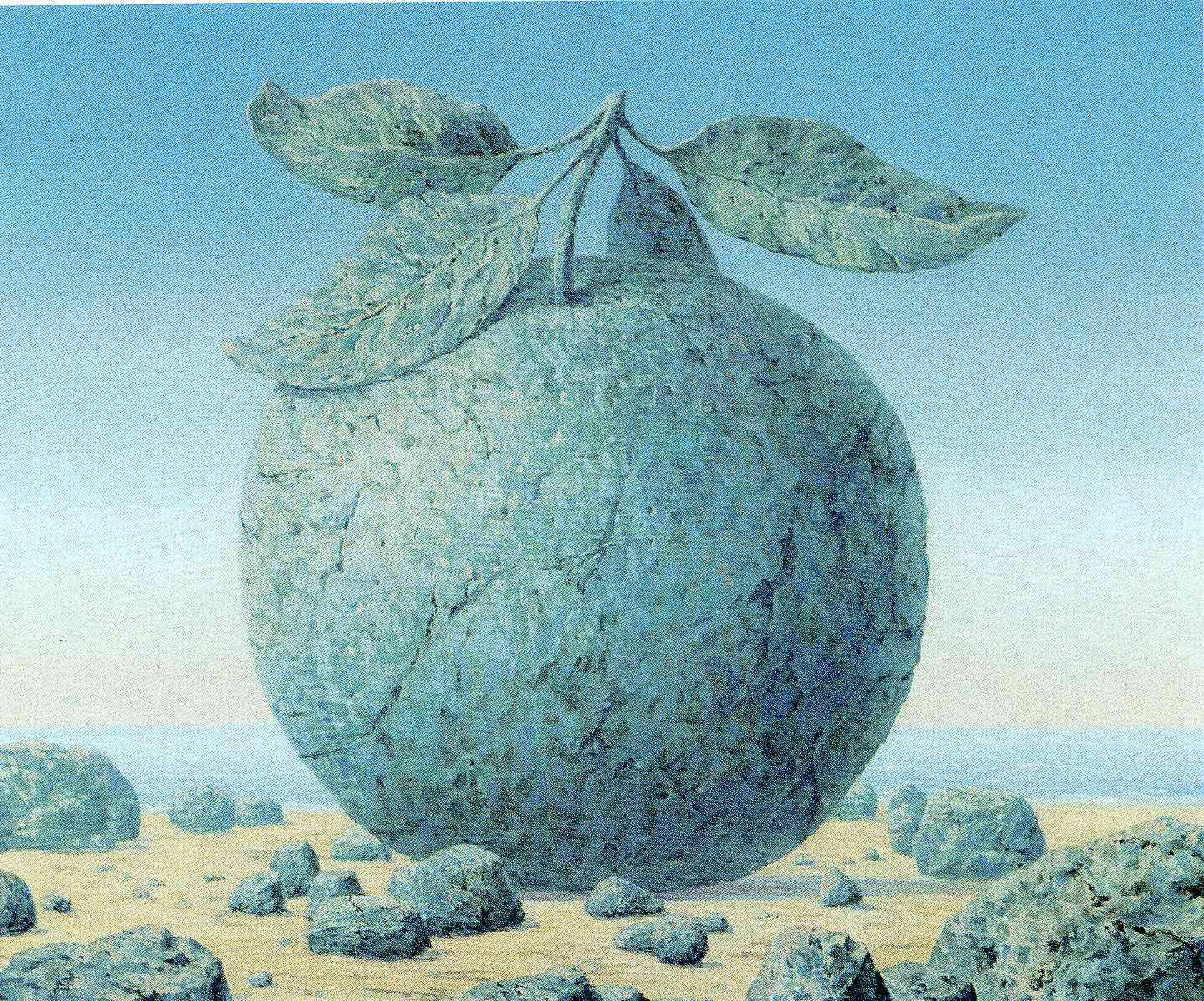This is an image of a large, surrealistic fruit—presumably an orange or peach—situated on a sandy beach. The fruit stands out due to its enormous size, dwarfing the surrounding rough, gray rocks. Its color palette includes tones of bluish-green, dark blue, yellow, and white, seamlessly blending with the rocky texture on the beach, as if the fruit itself is carved from stone. The fruit features a stem with four leaves, which also share the same rocky, artistic interpretation. Behind this giant, rock-like fruit, an ocean stretches to the horizon, with a sky that transitions from a light blue near the horizon to darker shades higher up, culminating in a faded blue tonal sunset with white and yellow hues. This entire scene, with its pixels and crevices in the fruit's surface, exudes a science fiction, computer-generated feel, enhancing the surreal and fantastical nature of the image.